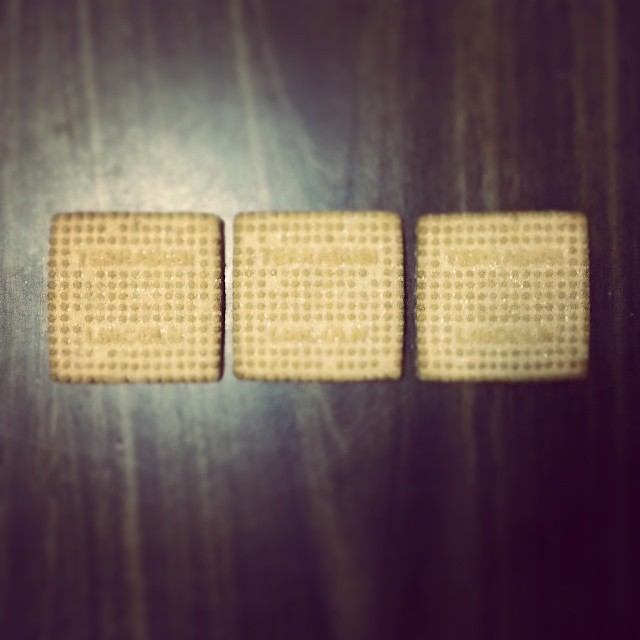A slightly out-of-focus, close-up color photo captures a dark wooden surface, resembling walnut, that serves as a tabletop or countertop. On this surface are three uniformly square-shaped objects, potentially cookies or crackers, aligned in a row. Each square is tan in color, featuring small, raised, round elements across their surface, and bears writing in two lines—one near the top and one near the bottom, although the words are not entirely legible due to the blurriness. A light source positioned behind the camera illuminates the scene, casting a soft glow around the squares and reflecting off the wood surface.